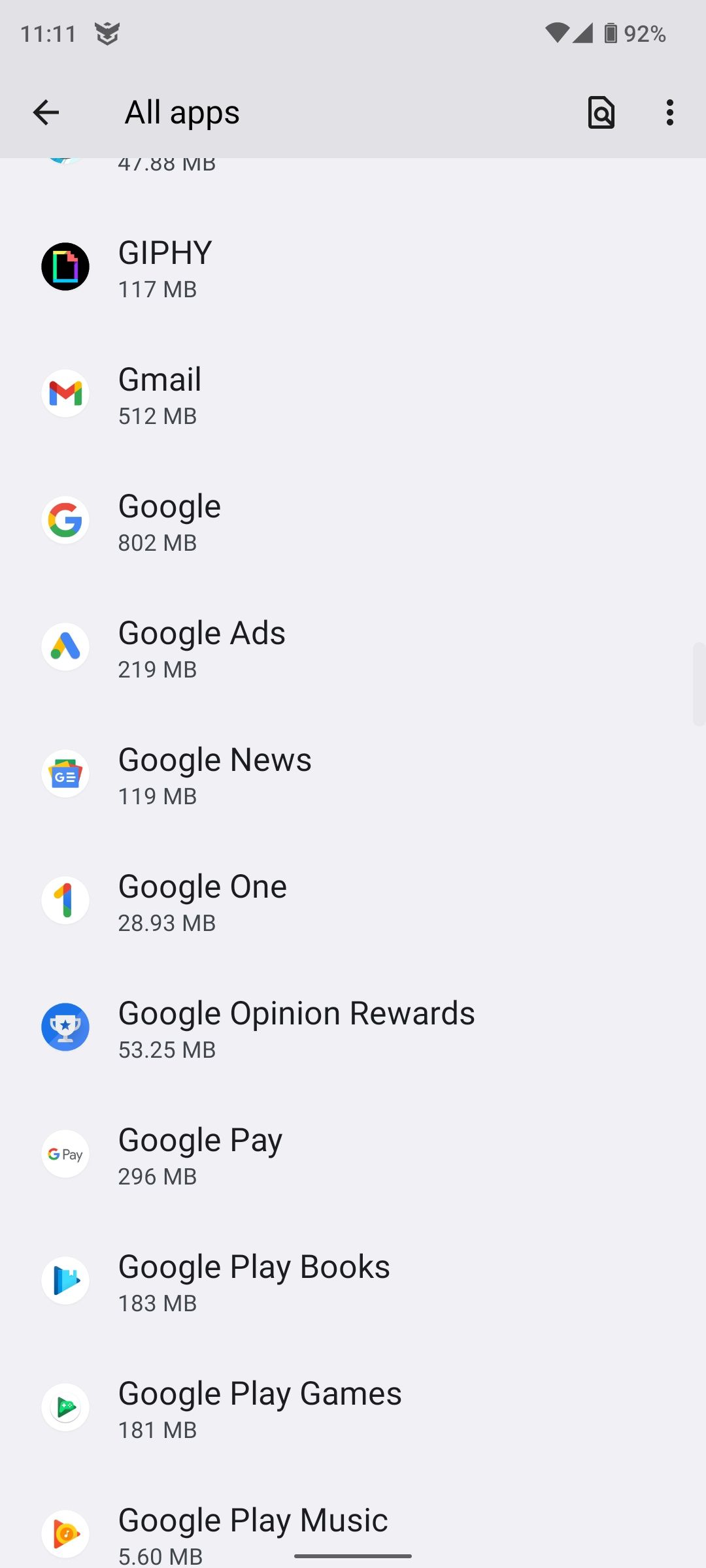The image captured from a cell phone display showcases a list of applications arranged in a vertical format. The screen's upper section features a darker gray rectangle where the time is displayed as "11:11" alongside a small icon. Moving leftward, there are indicators for Wi-Fi signal, a triangle symbol, and a battery icon showing a 92% charge.

Beneath this upper section, a centered title reading "All Apps" is accompanied by a left-pointing arrow on its left, suggesting a navigation option, and a paper icon with a corner folded on the right. At the far right, three vertically aligned dots indicate additional options or settings.

As you scroll down past the header "All Apps," a semi-obscured app appears behind it. Below this, individual apps are listed with their names and sizes. Notable apps include Giphy, consuming 117 MB, and Gmail with a size of 512 MB. Other visible apps include Google, Google Ads, and Google News, among others, populating the rest of the screen in a continuous downward listing.